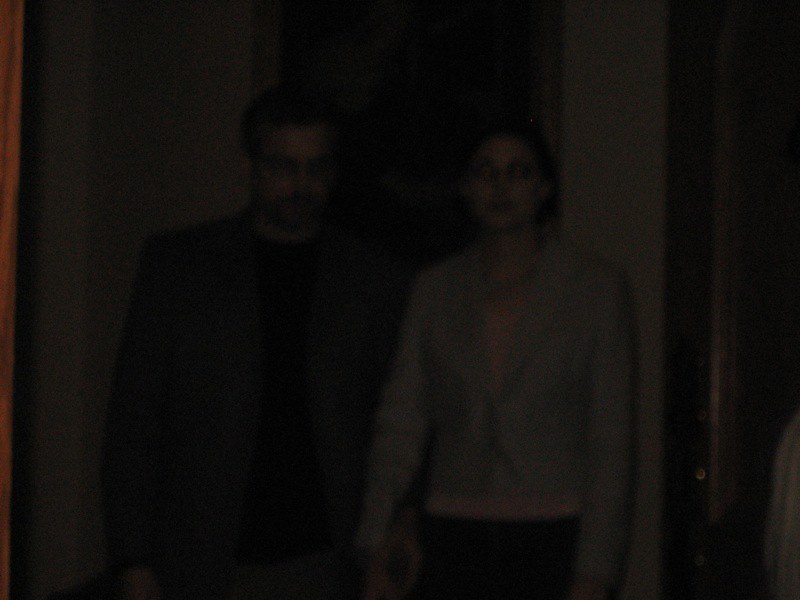In this image, we observe a heavily blackened and grainy photograph, possibly taken in a dark room or heavily filtered. The image vaguely reveals two individuals standing side by side, facing forward. Visible from the upper thigh upwards, the person on the right appears to be wearing a lighter-colored jacket with long sleeves and a shirt underneath. The jacket features a collar that extends from around the neck to mid-chest. The individual on the left, who seems to have short dark hair, is dressed in dark clothing, though the exact style or whether it is a one-piece or two-piece outfit remains indiscernible due to the extreme darkness and graininess of the photograph.